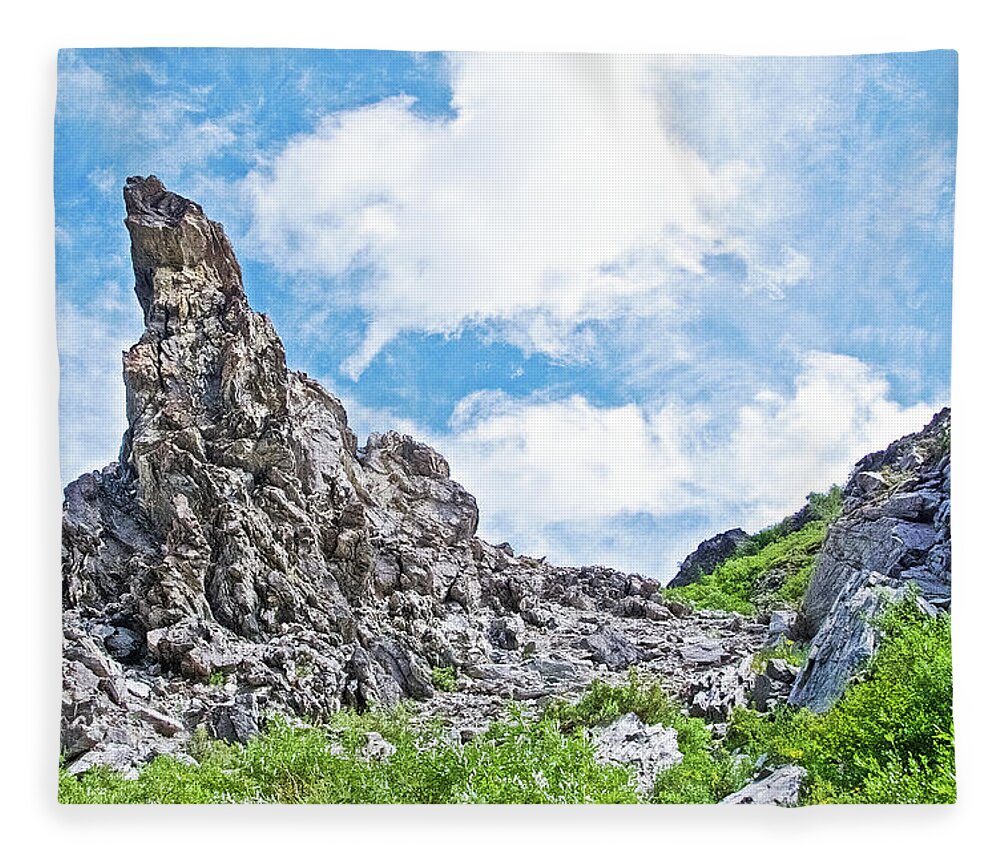This photograph captures the rugged beauty of a hillside or small mountain summit on a bright, sunny day. The image showcases a jagged, rocky formation, predominantly gray and dark gray in color, rising to the left side of the photograph. Interspersed among the rocks are tufts of vibrant green grass and low-lying leafy shrubs, giving a sense of lush but wild terrain. The rocky area extends across the bottom of the picture, with a path of flat rocks visible in the center, surrounded by the green foliage.

The sky, painted a stunning baby blue, hosts a scattering of big, fluffy white clouds, adding depth and contrast to the scene. This canvas-like photograph, complete with visible gray grid marks, accentuates the natural texture of the rocks and greenery, giving the impression of a photograph imprinted on needlepoint fabric. The overall atmosphere suggests a spring or summer day, providing a snapshot of nature's raw, unyielding yet beautiful landscape.